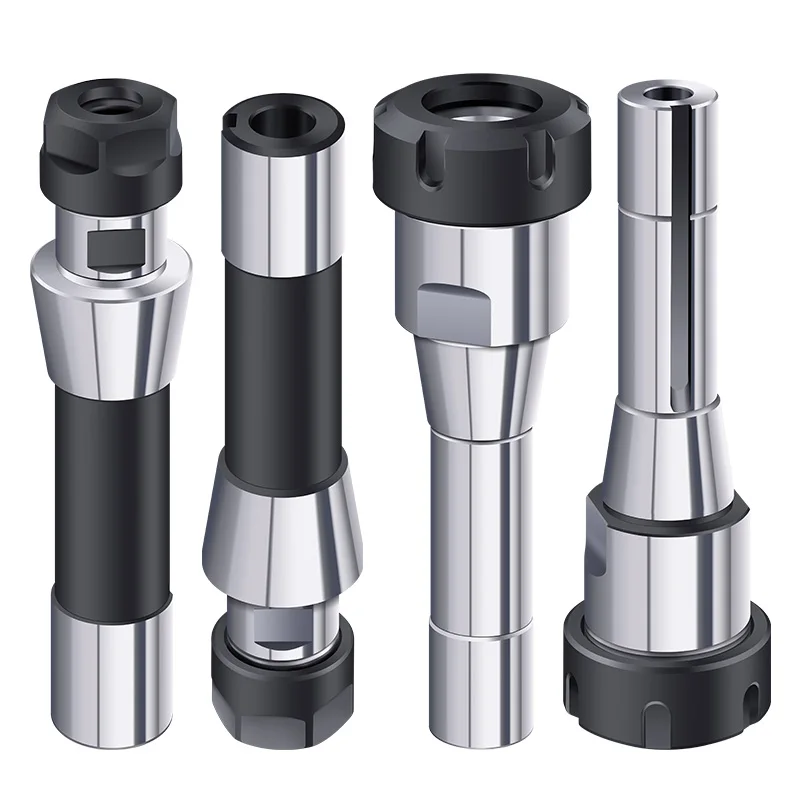The image features a detailed digital rendering of four metallic cylindrical structures, likely tools or tool add-ons, aligned side-by-side. Each object primarily exhibits a silver metallic body, with the first two cylinders from the left including black rubber grips around their centers. These cylindrical structures, which might be made from stainless steel, feature black end pieces that appear designed to be tightened or attached to a drill piece. The ends vary in size, with the first two cylinders having smaller end pieces compared to the slightly larger ones of the remaining two. Each structure also includes a dark gray or black cap, possibly covering a lens or similar component, suggesting a functional purpose possibly related to drilling or bolting. Despite their appearance akin to mini flashlights or bolts, the exact function remains unclear.